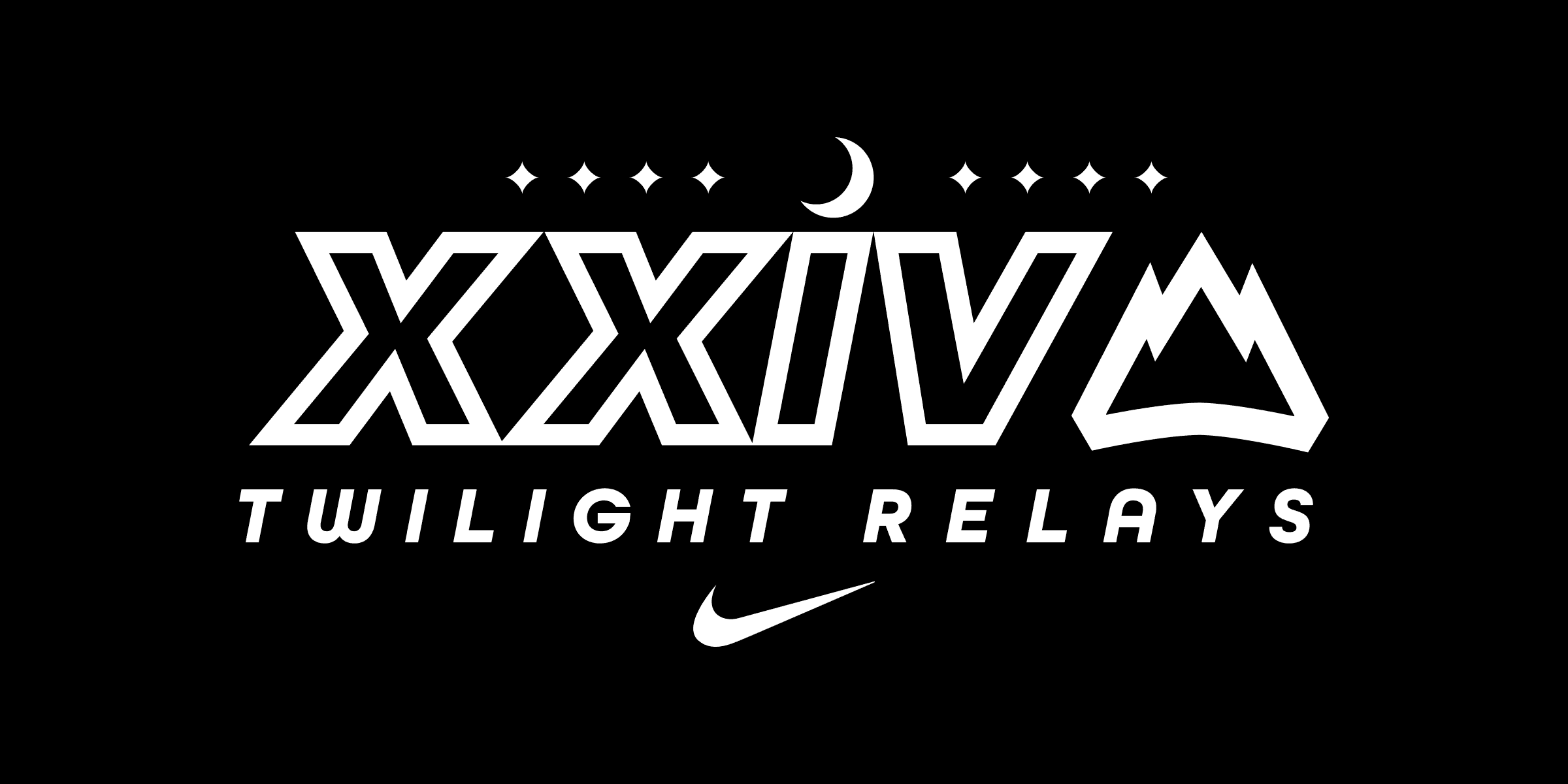The image is a digital drawing with a completely black background and features prominently white elements. At the top center, there is a stylized crescent moon flanked by four diamond-shaped stars, all in white. Below this celestial arrangement, large bold white letters spell out "XXIV." To the right of these letters is an outlined mountain range with three sharp peaks, also in white. Underneath the mountain range and extending across the width of the image, the text "twilight relays" is written in smaller white letters. Centered at the bottom of the image is the iconic Nike swoosh, also in white, suggesting sponsorship or branding. This minimalist design appears to be promotional artwork, possibly for a Nike event or product related to the "twilight relays."